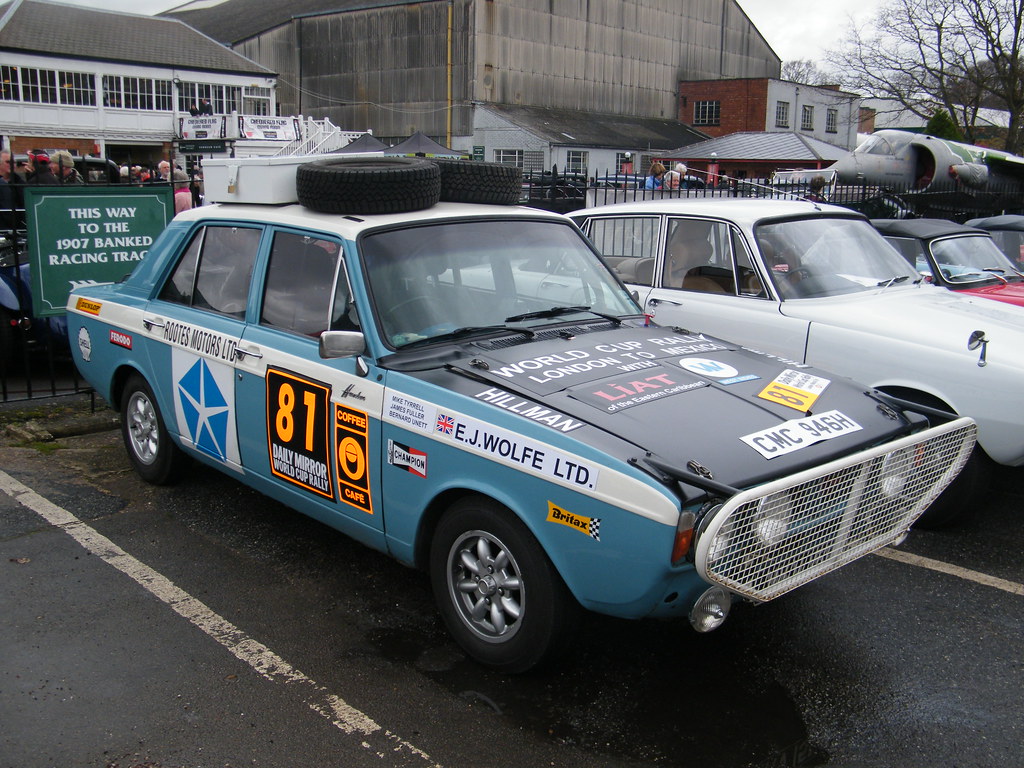The image captures a vibrant scene at a car meet set in a parking lot of an industrial area, featuring an array of vintage race cars and an aircraft. Dominating the center is an evocative rally car from the early 1980s, painted in a striking combination of blue with a white stripe along the side and a distinctive black hood. The car is adorned with various logos and text, including a prominent black box with yellow numbers '81' and white text that reads “Daily Mirror World Cup Rally.” Additional decals include “EJ Wolfley LTD Latte CMC 946H” and a Shell logo amongst others. Notably, the car is equipped with two spare tires and a toolbox on its roof, as well as a protective grate over the headlights. 

Flanking this central car to the right is an older white sedan, and adjacent to it, a red car. In the backdrop, you can discern a Harrier Jet meticulously parked, suggesting the presence of a museum or exhibit. The setting is further textured by a variety of structures: a gray cement building with an attached shed, a warehouse with numerous windows and a black roof, and distant small houses. People are scattered in the background, indicating a bustling gathering. Ornamental details such as fencing and trees interject, while the distant mountain and white sky frame the scene, capturing a lively and nostalgic moment.